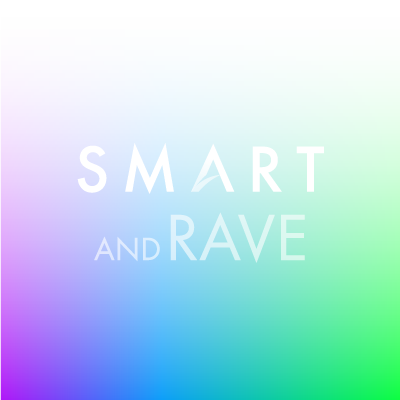The image showcases a vibrant gradient background that seamlessly transitions left to right from violet to blue to green, while also fading from a darker hue at the bottom to a lighter shade at the top, almost reaching white. In the center of this colorful backdrop, the words "SMART" and "RAVE" are prominently displayed in capital white letters. The "A" in "SMART" features a unique design: rather than a standard horizontal crossbar, it has a artistic diagonal swoop that extends from the bottom left upward to the middle of the right leg. The text appears slightly transparent, harmoniously blending with the gradient background.